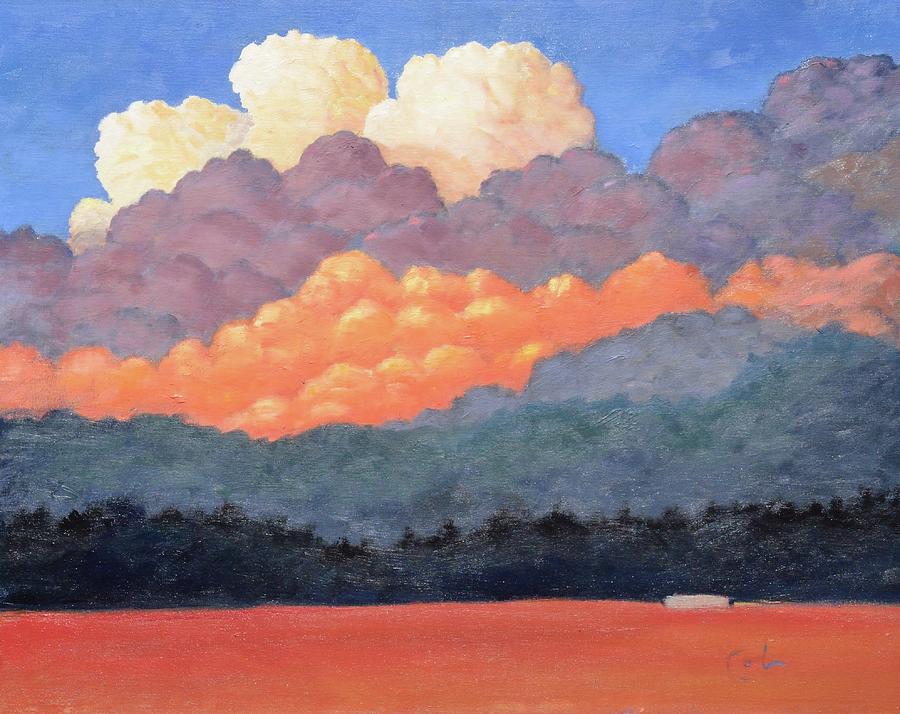The image depicts a vividly colored painting of a surreal landscape. The sky is a bright shade of blue, filled with clouds arranged in distinct layers that vary in color. At the top, three white, fluffy clouds float, followed by a layer of dark charcoal-gray clouds. Below them, a sequence of clouds transitions into an orangey-peach hue, before shifting again to a dark gray. Beneath the sky, the horizon features a row of trees rendered in a stark black silhouette. The ground, or field, diverges from the typical green, appearing instead in a striking shade reminiscent of strawberry lemonade. This reddish-pink field adds to the painting's dreamlike quality. With an undercurrent of intense, vibrant colors—ranging from burgundy and purple to blue-green—the artwork portrays a fantastical, almost otherworldly scene, underscoring its nature as a meticulously crafted painting rather than a depiction of a real landscape.